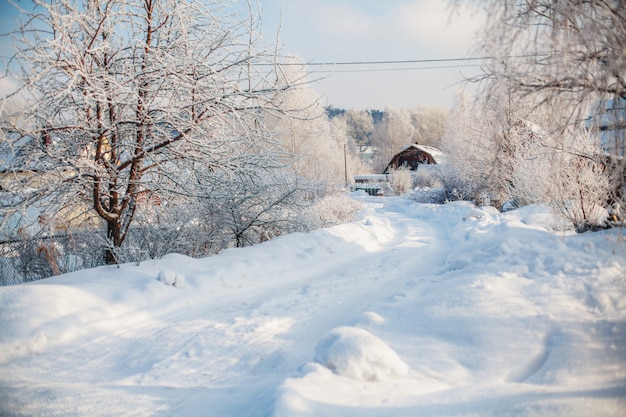This photograph captures a tranquil winter scene in the countryside, featuring a snow-covered back road flanked by barren, snow-laden trees. The road appears to have been plowed, with noticeable mounds of snow on either side, yet still shows tire tracks as evidence of recent travel. To the left, there is a tall tree covered in snow with a chain-link fence at its base. On the right, another tree with elongated, snowy branches mirrors the wintry ambiance. Overhead, power lines stretch horizontally across the blue sky dotted with light clouds, contributing to the serene atmosphere. In the background, a dark brownish-red barn with a snow-covered roof stands out, partially obscured by more snow-capped trees. The crisp air and the silence of the snow create a picturesque, almost photorealistic quality to this winter wonderland, accentuated by the bright sunlight reflecting off the icy surfaces.